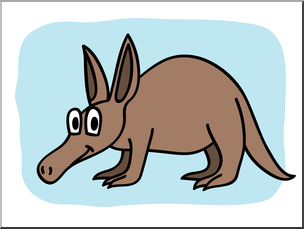The image showcases a cartoon-style illustration of a cheerful brown creature, reminiscent of an aardvark, set against a color-blocked background with white and light blue sections. The setting suggests an outdoor scene. The central figure, which has an oval-shaped body, features expressive black eyes within larger white ovals and a long snout with two nostrils. Its head is tilted downward towards the bottom left corner, smiling cheerfully. The creature has tall, pointy ears with a darker brown inner layer and stands on four legs with tapered, pointy toes. A long tail extends from its body, rounding out this charming and whimsical depiction.